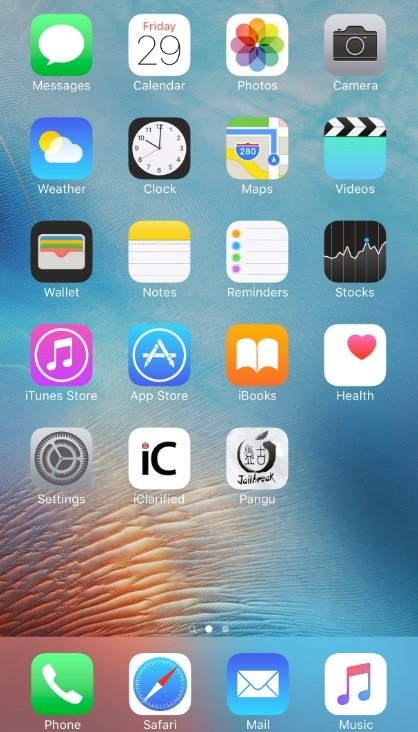A detailed screenshot of a mobile phone's home screen featuring a captivating abstract blue wallpaper. The wallpaper has a texture reminiscent of wet sand at the bottom, offering a visually engaging background. Prominently displayed are several rows of app icons, organized as follows: 

- **Top Row (left to right):** Messages, Calendar, Photos, Camera.
- **Second Row:** Weather, Clock, Maps, Videos.
- **Third Row:** Wallet, Notes, Reminders, Stocks.
- **Fourth Row:** iTunes Store, App Store, iBooks, Health.
- **Fifth Row:** Settings, iClarified, Pangu.

At the bottom, a translucent bar hosts four essential apps:
- **Left to right:** Phone, Safari, Mail, Music.

Just above this bar, three small dots indicate the presence of additional home screens for navigation.